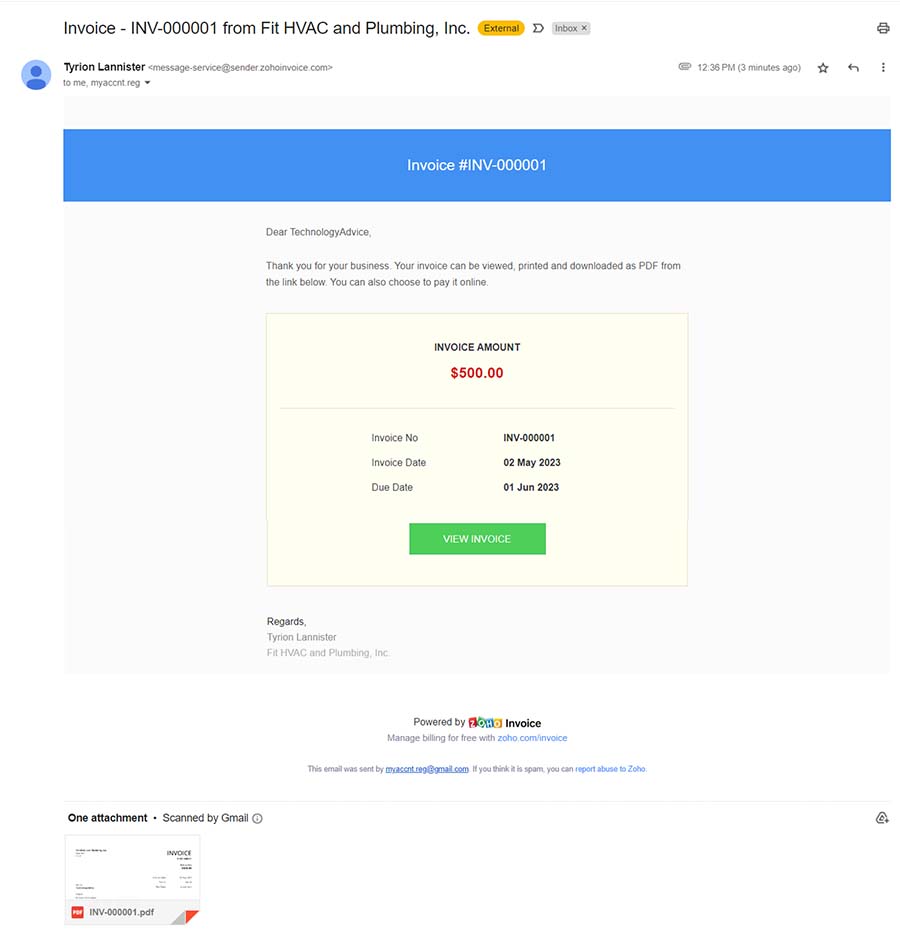A detailed screenshot of a recently issued plumbing invoice totaling $500 (colloquially referred to as "doll hairs" by the viewer's girlfriend). The invoice, with a blue header and white background, was sent just three minutes ago as an email. The invoice was issued on May 2nd and has a due date of June 1st. It reflects the high costs often associated with plumbing services. The invoice is signed off by Tyron Lansing with the note, "Regards."